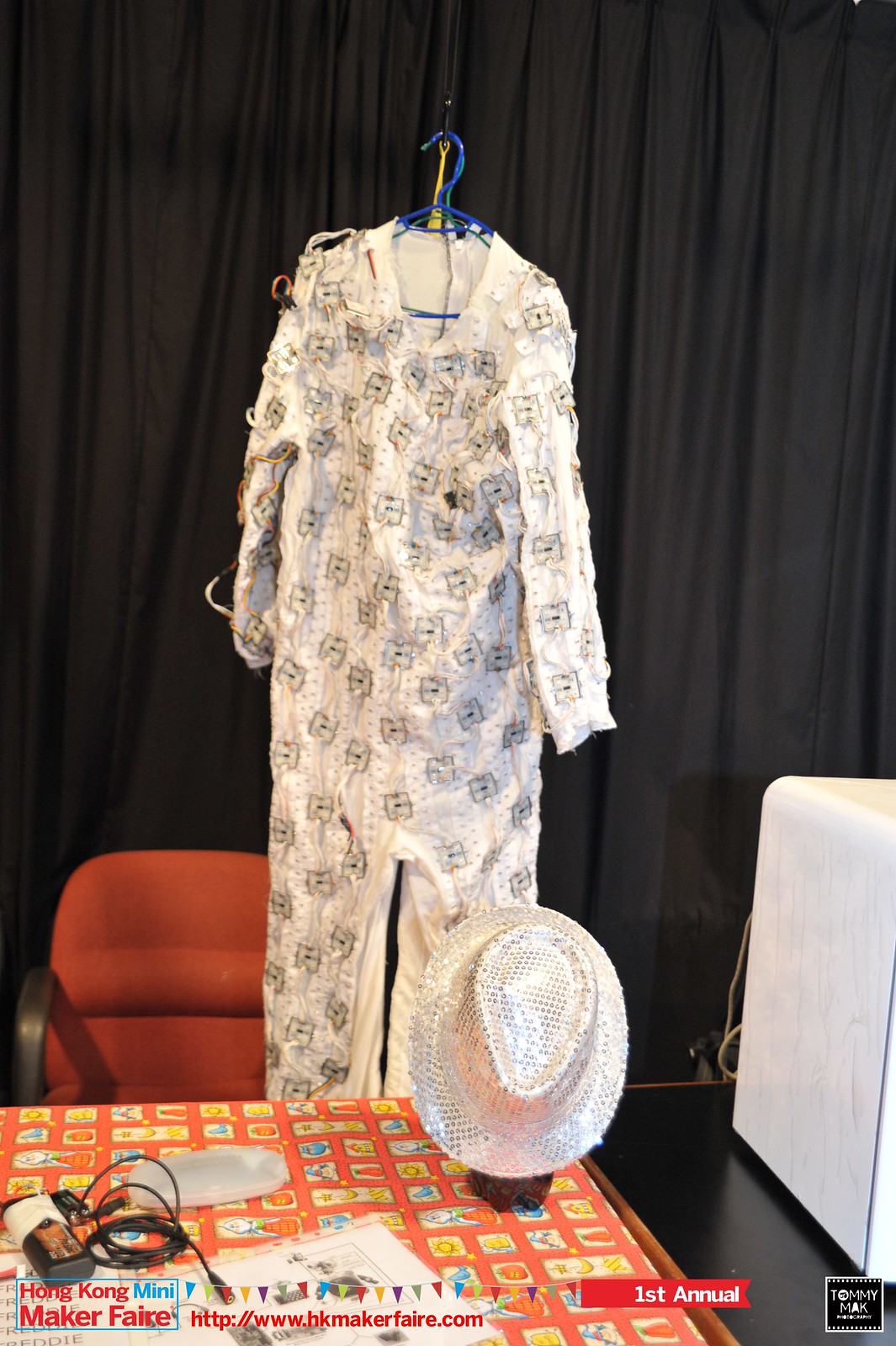The photograph captures an indoor setting, showcasing a detailed white onesie outfit adorned with square patterns featuring black minus symbols. This outfit is hanging from a blue hanger, which is suspended by a black hook from the ceiling. In front of the outfit, there is a table covered with a multicolored, patterned cloth featuring yellow, blue, and orange designs. Resting on the table is a distinctive white cowboy hat, decorated with shiny specks and diamond-like patterns. Additionally, the table holds various items including a charger, an eyeglasses box, and some papers. To the side of the table is an orange cushioned chair. The background features black curtains. At the bottom of the image, there is a blue-bordered box with the text "Hong Kong Mini Maker Faire" and the website "http://www.hkmakerfaire.com," along with celebratory ribbon designs. Towards the right, a red horizontal box reads "First Annual," and in the bottom right corner, a black square with white borders displays the text "Tommy Mac."